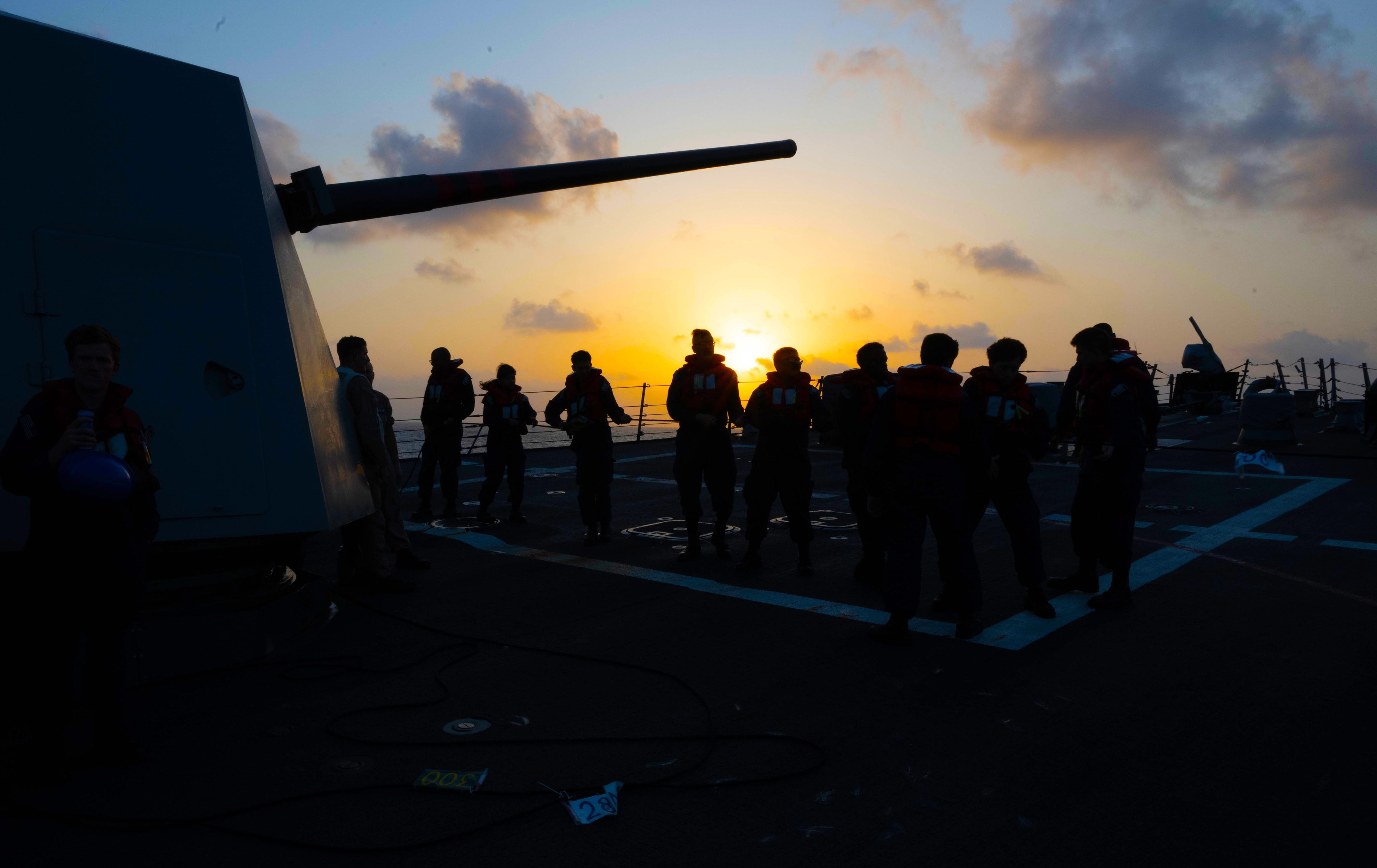In this striking photograph, the sun is setting, casting a mesmerizing palette of yellows, blues, and oranges across the sky, with grey clouds lit up by the glowing sunset. The image captures a group of ten silhouetted figures standing on what appears to be a boat or floating cargo ship, with their backs to the camera, gazing towards the horizon. The ground they stand on is black, marked by a white rectangle and some barely discernible numbers, suggesting the outline of a landing pad. Encircling them is a fence that blends into the dark surroundings. On the left side of the photo, a long, cylindrical, cannon-like item juts out from a structure, adding a sense of intrigue to the scene. Despite the darkness enveloping the image, the vivid colors of the sky create a captivating contrast, highlighting the serene yet solemn mood of the moment.